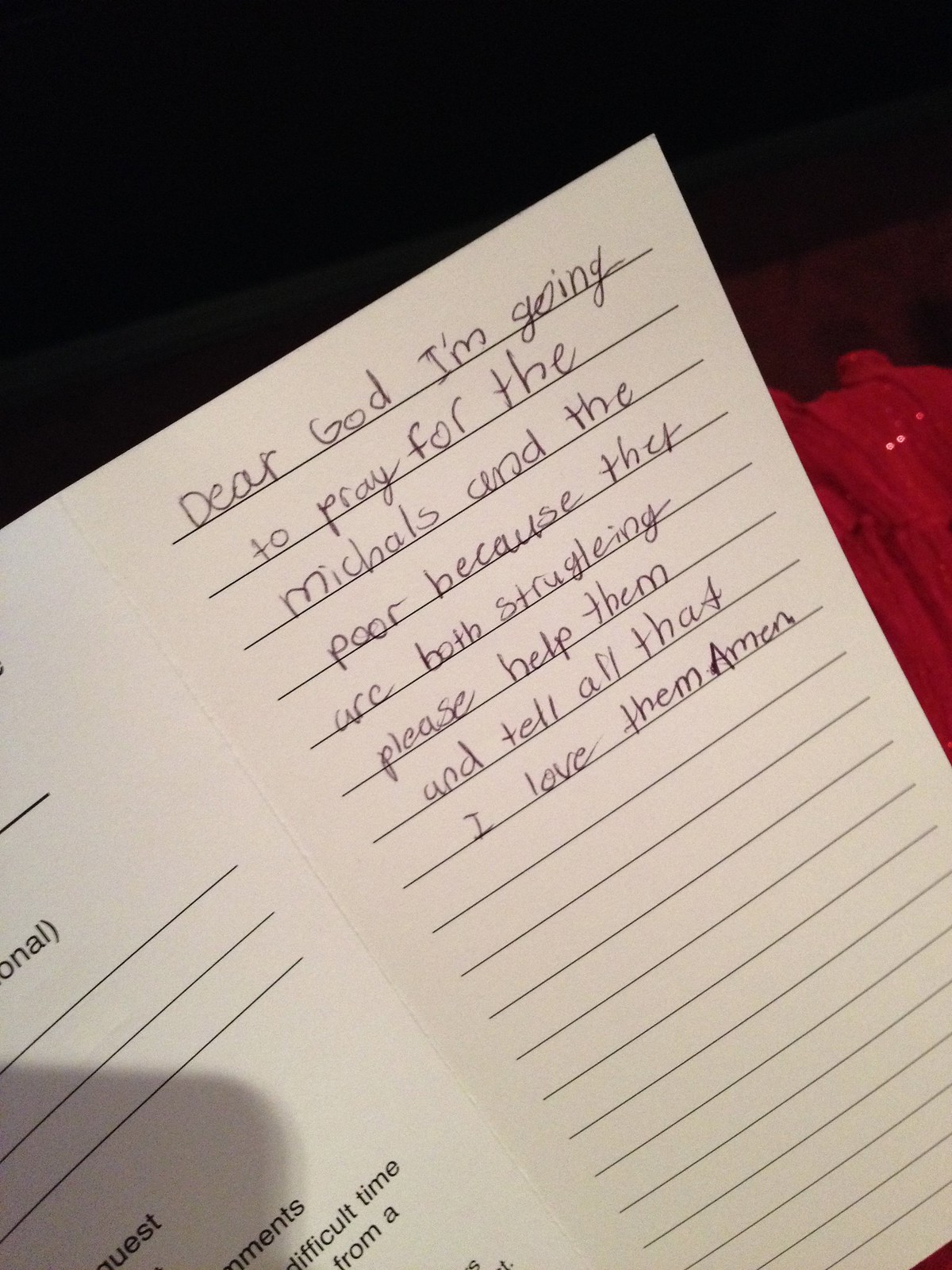This color photograph, taken in portrait orientation, captures an open white-lined prayer journal. On the right-hand page of the journal, written in black ink, is a heartfelt handwritten message that reads, "Dear God, I'm going to pray for the Michaels and the poor because they are both struggling. Please help them and tell all that I love them. Amen." The text is set against a backdrop of several blank lines, awaiting further entries. Opposite this, on the left page, partial printed text is visible, with words like "difficult time" hinting at the context of the writing. The journal rests on a surface with a red cloth to the right, contrasting against the predominantly black background. Light entering from an angle casts a slight shadow on the book, adding depth to the scene. The pages are slightly tilted from the top left to the bottom right, emphasizing the personal and intimate nature of this reflective moment.